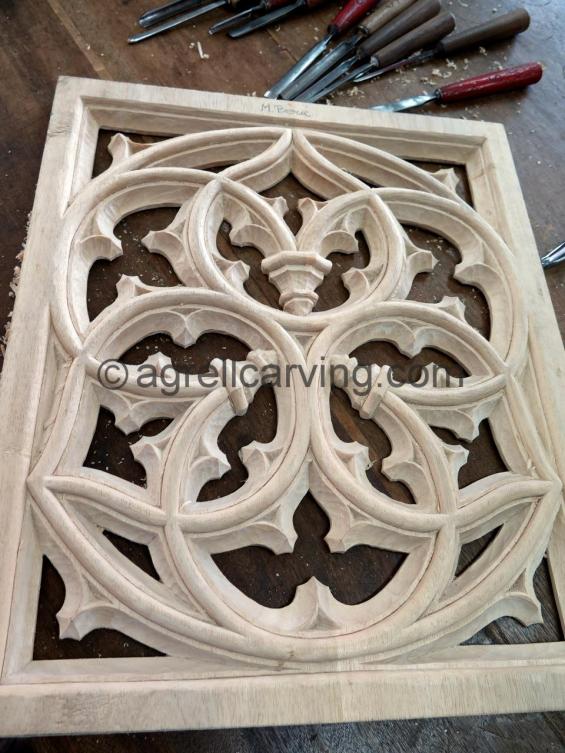The photograph features an intricately carved wood art piece resting on a dark brown desk. The artwork, a rectangular frame carved into a pattern of overlapping circles and rings that almost resemble leaves, showcases an artistic design with parts elegantly cut away. The light tan wood contrasts with the workspace, which is strewn with wood shavings, indicating recent activity. Positioned above the carving are various chisels with red, brown, and black handles, tools used for the detailed craftsmanship. The image was taken from a lower angle in front of the piece, partially obscuring the bottom corners while displaying the top corners clearly. In the center of the photograph, a watermark reads "© agrellcarving.com," adding a signature touch to the piece.